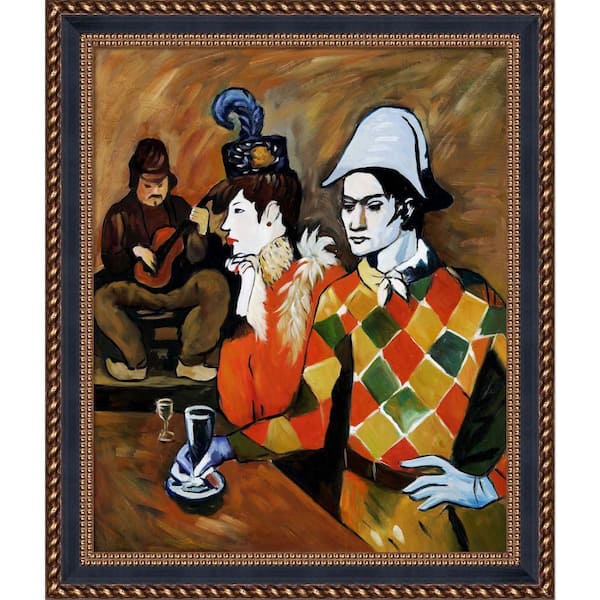This is an oil painting featuring three distinct individuals, all with very white skin, set against a predominantly brown-toned background. The painting is framed in an ornate, alternating gold and black wooden frame with raised, embossed patterns on the gold sections. In the foreground, two people are standing at a wooden table that occupies the bottom left corner of the canvas, each with a drink resting on the table.

The closest figure, a striking character reminiscent of a Joker, is adorned in a diamond-patterned sweater of red, green, and yellow, complemented by a white neckerchief. His black hair is topped with a white and black Napoleonic hat, and he sports white gloves. His pose is confident with one gloved hand rested on the bar or table.

To his right stands a woman in a vibrant red shirt, accentuated by a white fuzzy scarf. Her brown hair is decorated with a brown hat featuring a blue feather and a flower, adding a dash of color. She wears an earring, and her ensemble radiates an air of vintage elegance.

In the background, adding a musical ambiance to the scene, is a man sitting on a chair, engrossed in playing a small guitar or fiddle. He wears brown pants and a dark brown shirt and hat, with a distinct mustache and goatee. His feet are notably turned outward, and his posture suggests concentration, emphasizing his role as a musician in this quaint, possibly bar-like setting.